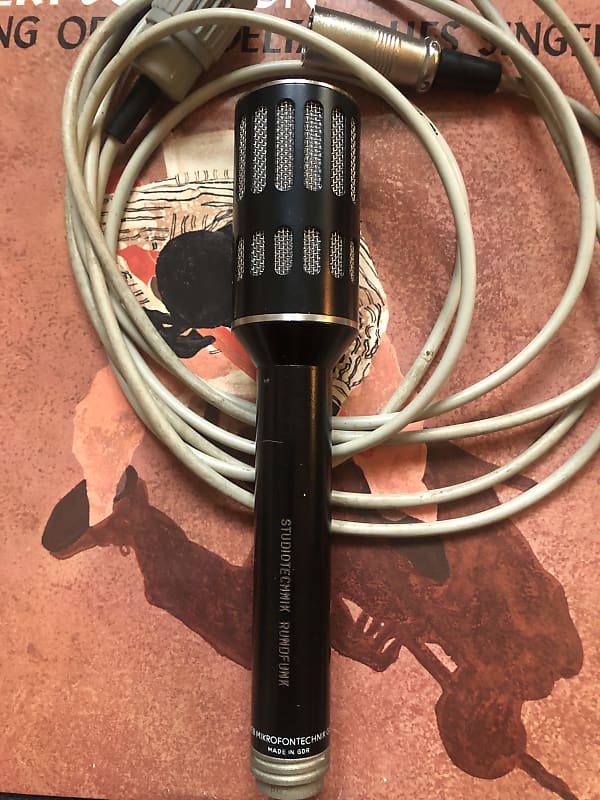The image displays a black, cylindrical microphone, prominently featuring the text "Studio Technic" and "Rund Funk" engraved vertically in grey. The microphone has a wider section at the top, which is adorned with oval-shaped holes revealing a steel mesh, indicative of its grill. At the bottom of the microphone, there is a visible metallic connector. Resting beneath the microphone is a coiled, beige microphone cable with metal ends, likely intended to connect to the microphone. The background appears to be an abstract illustration or the cover of a book, predominantly red with texture, featuring what seems to be an image of a person wearing a red shirt. Scattered white and dark spots add to the background's textured appearance. Faint, hard-to-read text is visible towards the top of the image. The overall scene suggests this could be a product listing photograph, possibly for a platform like Craigslist or eBay.